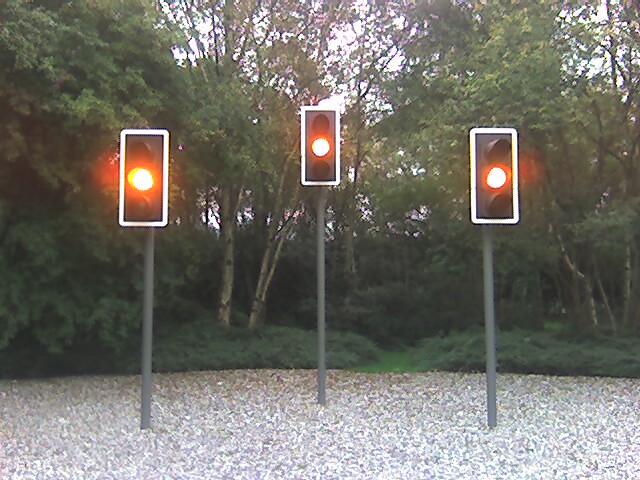In this captivating outdoor scene, the foreground is dominated by three thin, gray poles, each topped with a traffic light. The lights are symmetrically aligned, forming a slight triangular formation. All traffic lights are illuminated with a yellow light, which gives off a reddish hue, subtly lighting up the surrounding area. The poles are planted firmly into a concrete surface that resembles a street, though the ground is also strewn with a thick layer of leaves in various shades of green, brown, and white, adding a natural texture to the scene.

Behind the traffic lights, the area transitions into a lush, wooded backdrop featuring tall, thick trees and dense bushes. The trees, with their towering presence and vibrant greenery, create a natural canopy, but there are glimpses of clear blue sky breaking through the foliage at the top of the picture. The scene blends the structured, urban element of the traffic lights with the serene, untamed beauty of the forest, resulting in a striking contrast. The interplay of light and color, especially the glow from the traffic lights, adds a captivating layer of depth to this intriguing image.